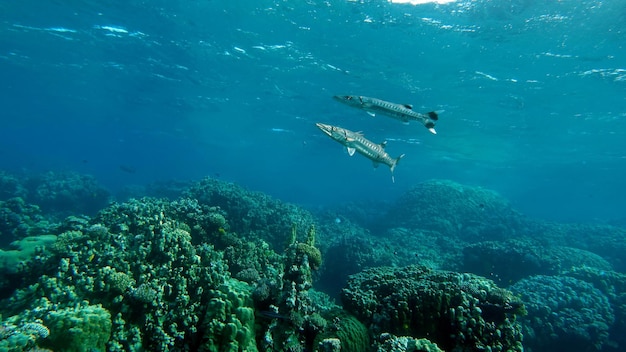This underwater photograph captures a spacious ocean scene with a gradient of vivid blues dominating the upper half of the image, highlighted by sporadic streaks of white light penetrating the water. The focal point is two medium-sized fish near the center. The foremost fish, positioned centrally with its head angled slightly upward to the left, boasts a silvery hue accentuated by subtle light-colored markings. It features a prominent fin atop its body, two fins underneath—one just behind its gill—and a tail trailing behind. The second fish, which is slightly darker and positioned slightly behind the first, mirrors the orientation with its head leftward and its body extending to the right. This fish's head is gray, and it sports a silver body with a distinctive black fin atop and a silver tail edged in black.

Beneath these swimming fish, the underwater terrain is a murky green, dotted with patches of algae, coral reefs, and some protruding rocks, providing a rich textural contrast to the blue expanse above. Amid the backdrop, the faint outlines of other distant fish are barely discernible, adding a sense of depth to the scene. The harmonious blend of blues and greens, coupled with the serene yet dynamic movement of the fish, encapsulates the tranquil beauty of the ocean's depths.